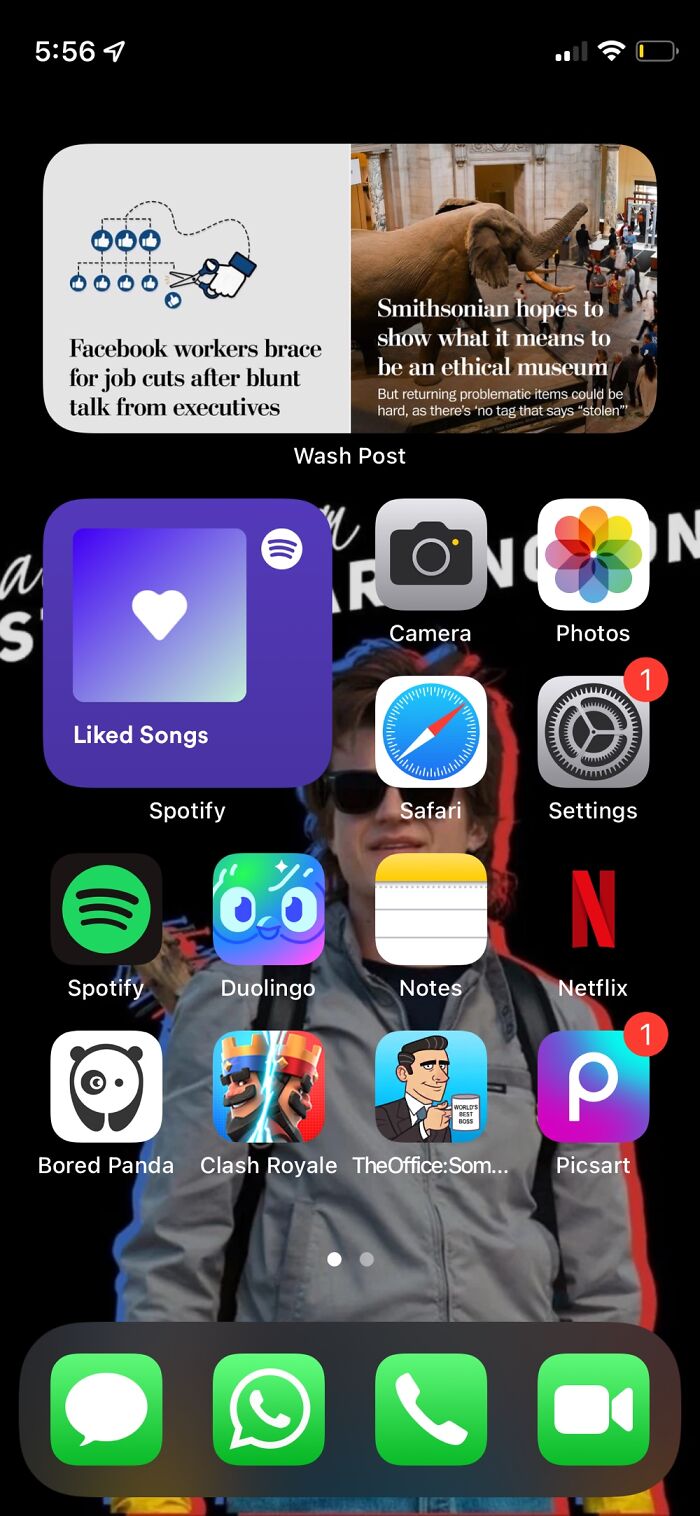The screenshot depicts a smartphone home screen featuring a minimalist black background adorned with an artistic image of a person with a striking red shadow. The screen is organized with various widgets and app icons. At the top, there's a widget labeled "Light Songs," followed by icons for Facebook, a work-related application identifiable as “Worker,” and the Smithsonian app.

Below these widgets, the screen shows a camera icon, along with the "Photo" and "Settings" apps. The next row includes icons for Safari, Notes, Netflix, The Office, an art-related app, and the game Clash Royale.

Further down, there are apps like Pork Panda, Spotify, and Duolingo. The layout continues with a noticeable section displaying green icon apps with white symbols, including Messages, WhatsApp, the Phone app, and FaceTime.

Overall, the screen presents a well-ordered collection of apps and widgets against a sleek dark-themed background, accentuated by the vivid red shadowed figure.